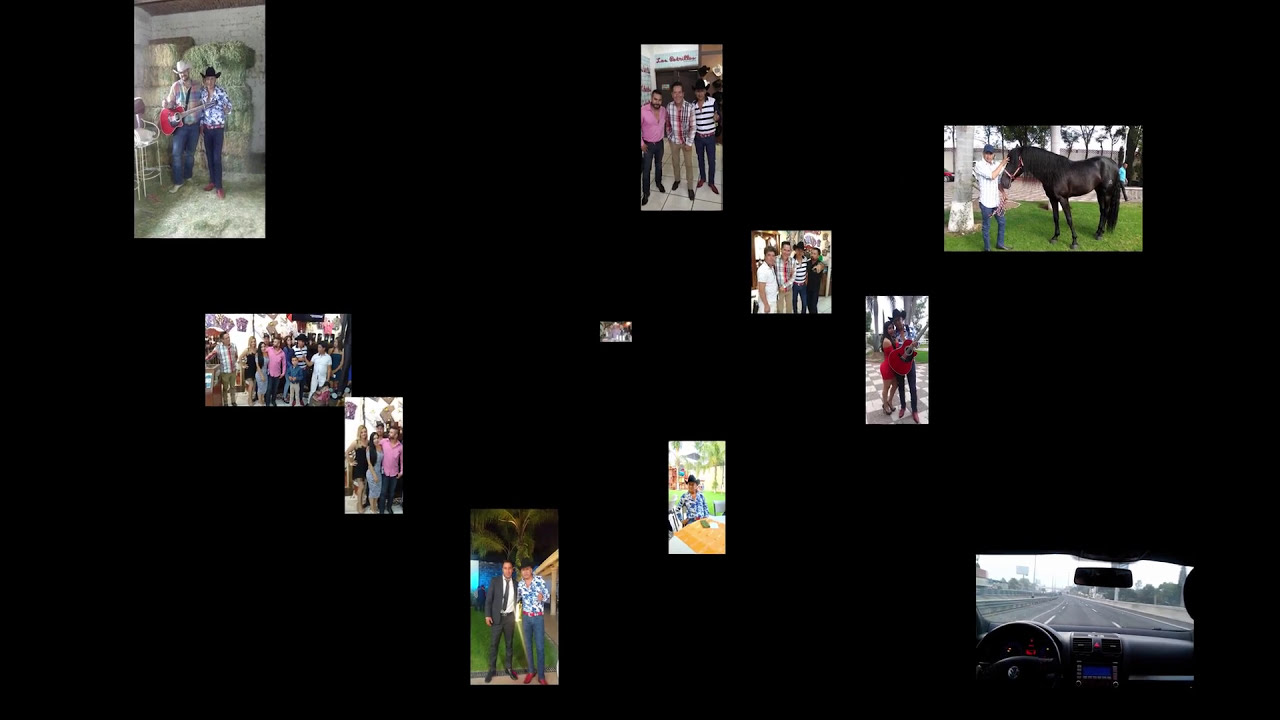The image features a collage of eleven distinct photographs, all arranged on a solid black background. Prominent among these are multiple group and individual portraits, with many subjects looking directly at the camera. Key highlights include a top-right photograph of a man petting a black horse on grass, and a bottom-right interior view of a car looking out onto a road. To the left, one image depicts a man with a guitar, giving off a cowboy vibe, standing next to another man. Below this are recurring characters, including a man in a pink shirt with his arm around a young lady, and two gentlemen—one in a suit jacket and another in a long shirt and red shoes—posing in front of a palm tree. Central in the collage, there is a picture of three individuals, and to the left, a group photo with some subjects appearing in close-ups beneath it. These images are eclectic, possibly from someone's personal collection, brought together into a random, yet cohesive layout on the dark background. The collage features a broad spectrum of colors including black, gray, green, red, blue, pink, purple, yellow, and tan.